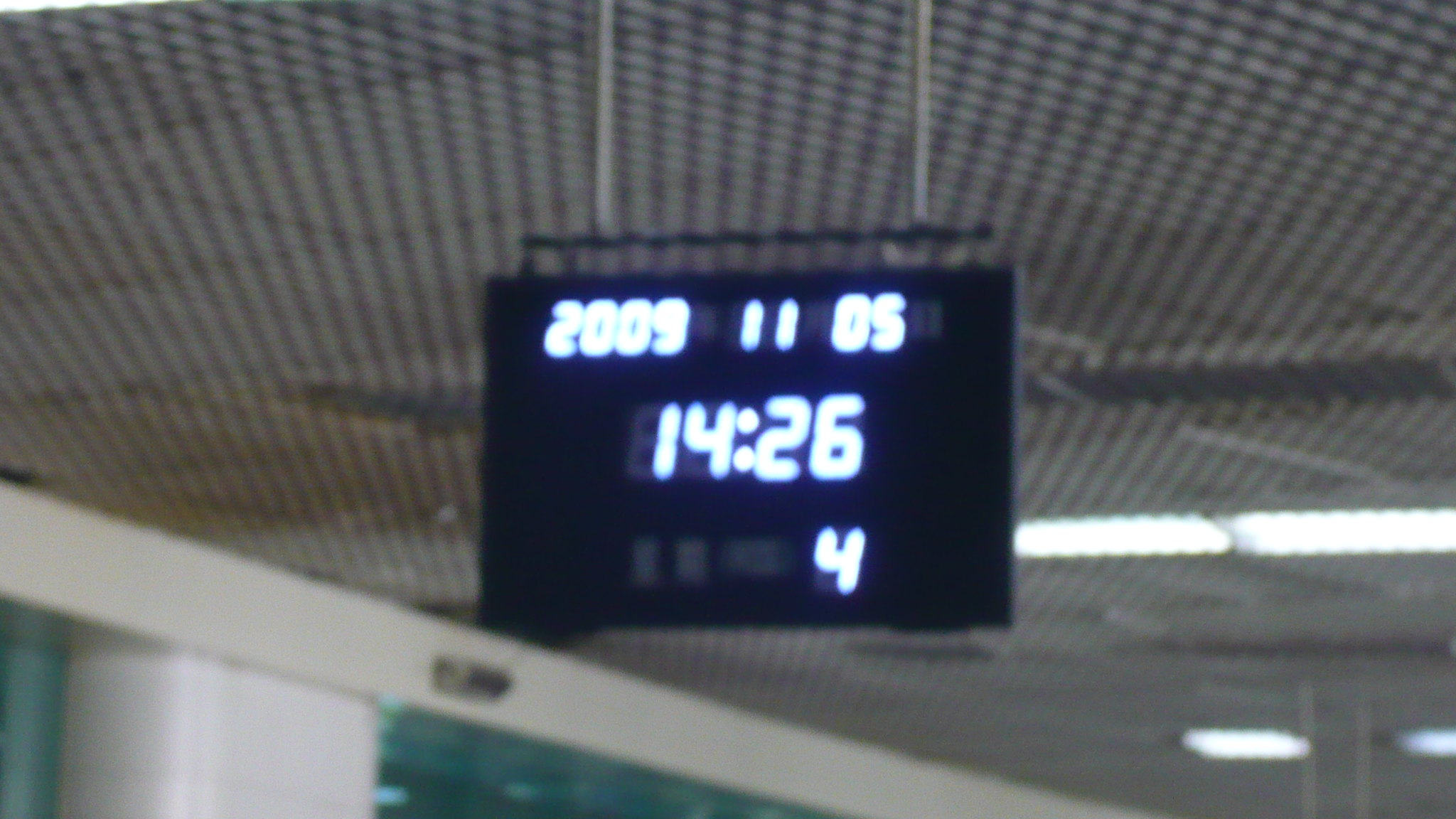A digital display sign, suspended from a light gray ceiling, features a sleek black background with crisp LED digits. Positioned at the top left corner of the screen is the year "2009". Adjacent to it, the numbers "11", "05", "14", "21", and "26" are sequentially displayed across the main section. The bottom right corner shows the number "4". Overhead lighting fixtures are faintly visible against the ceiling. To the left of the display, a section of a white wall and a white pillar come into view, while a transparent glass wall stretches further to the left. The monochromatic tones and modern elements of the scene offer an ambience of contemporary sophistication.